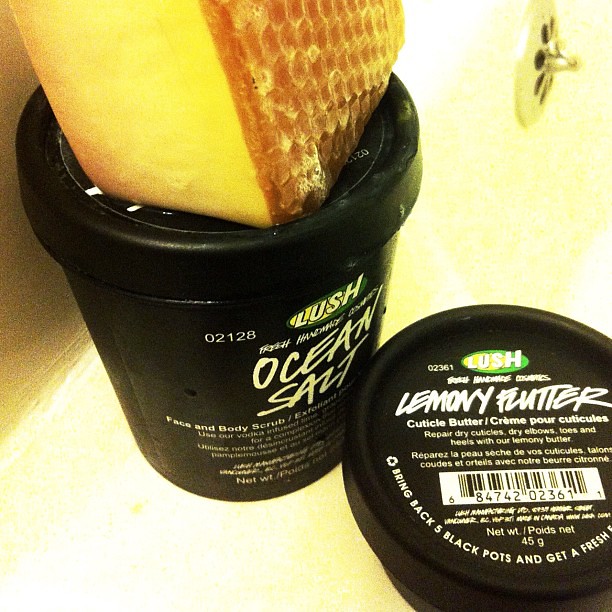The image depicts a dimly lit, amateur-style Instagram photo taken from above, showcasing two black cosmetic containers on the edge of what appears to be a white bathtub or sink. The smaller container in the foreground is labeled "Lemony Flutter" with additional text in French, describing it as "Cuticle Butter" for repairing dry cuticles, elbows, and toes. The label also includes a note about returning five black pots to receive a fresh product. The larger container behind it displays the "Lush" logo with the name "Ocean Salt," a face and body scrub, printed in white letters. Atop the "Ocean Salt" container sits a bright, waxy yellow and orange square, resembling a honeycomb-textured sponge. The overall background is predominantly white, highlighting the black containers and their distinct labels.